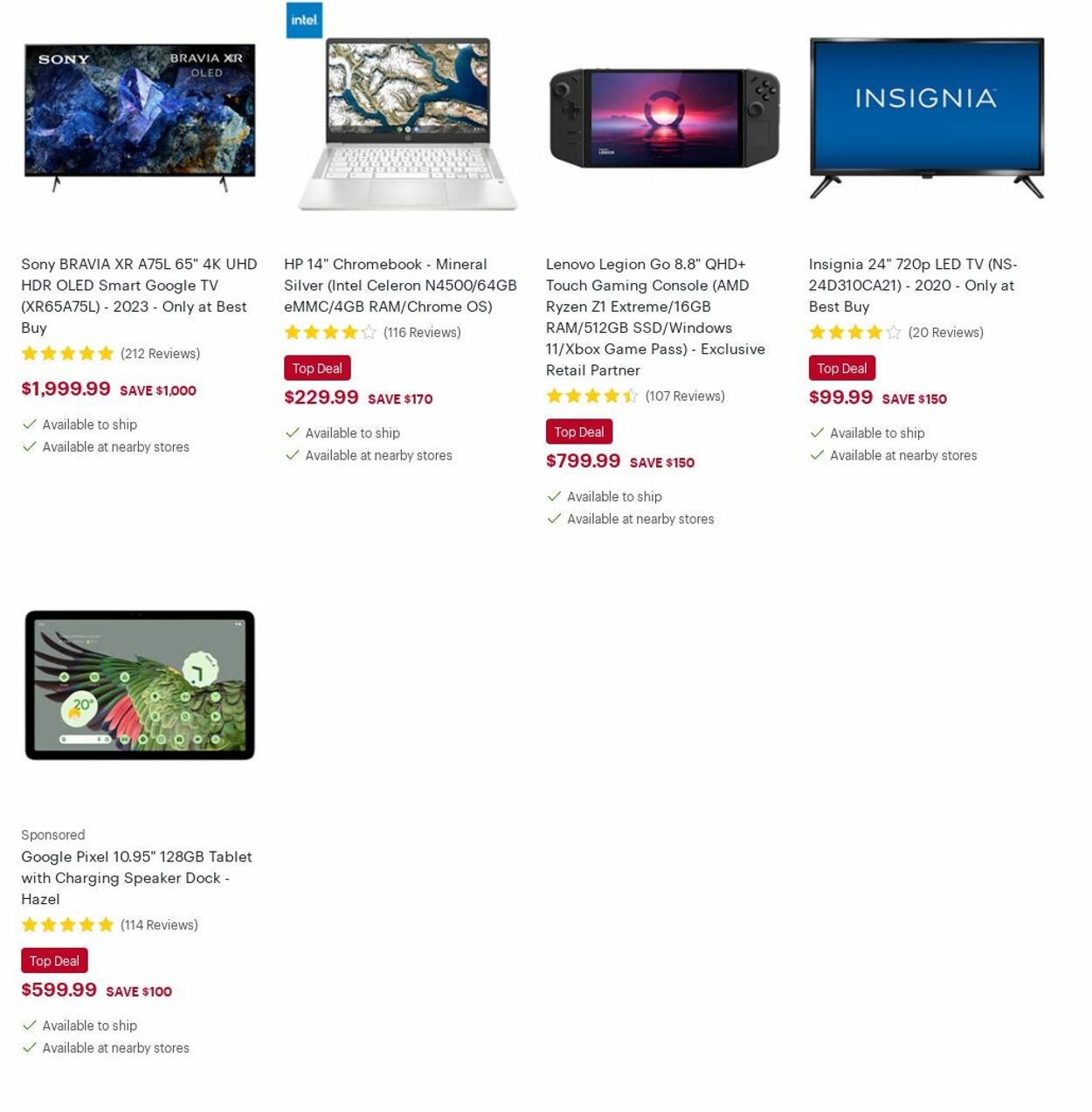The image displays a variety of electronic items with their respective prices prominently highlighted. A large, high-definition TV is priced at $1,999.99, showcasing a sleek design. Next to it is a compact and efficient laptop available for $329, ideal for everyday computing needs. A premium Bluetooth speaker, known for its superior sound quality, is listed at $799. Another TV, more budget-friendly at $99.99, offers an affordable option with essential features. Finally, an iPad is priced at $599.99, offering a perfect blend of portability and performance for on-the-go productivity and entertainment.